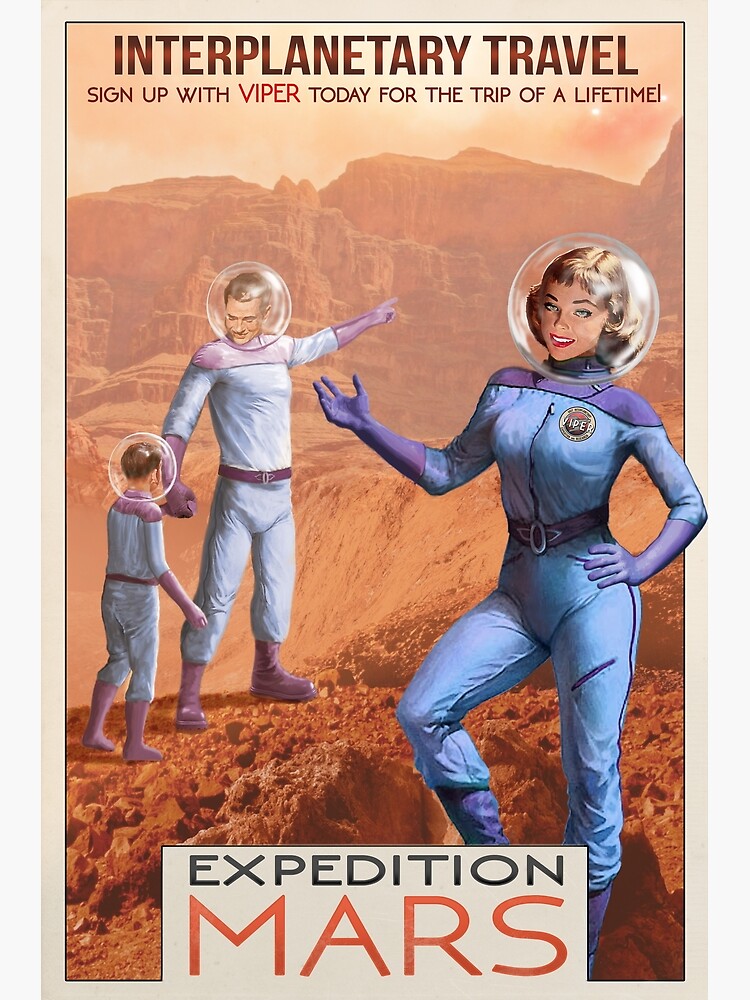The image is a meticulously detailed travel poster advertising "Interplanetary Travel" with the catchy slogan, "Sign up with Viper today for the trip of a lifetime." The text "Interplanetary Travel" is prominently displayed at the top in bold black letters against a red stripe, while "Viper" stands out in solid red text. At the bottom, the words "Expedition Mars" are featured, with "Expedition" in black and "Mars" in vivid red font.

The poster portrays a family—mother, father, and son—standing on the Martian surface, easily recognized by the red dirt and otherworldly landscape, including red mountains and a sky featuring at least two small moons. All three individuals are dressed in blue spacesuits with purple collars, gloves, and boots, and clear dome helmets. The father, positioned to the left, points towards the upper right corner of the image while holding the son's hand. The son, facing the same direction, is standing next to him. To the right, the mother strikes a confident pose with her left hand on her hip, her right arm bent with the palm up, and her right knee slightly raised. She gazes directly at the viewer with a smile, her head slightly tilted. The overall scene exudes an adventurous spirit, inviting viewers to imagine themselves embarking on an extraordinary journey to Mars with Viper.